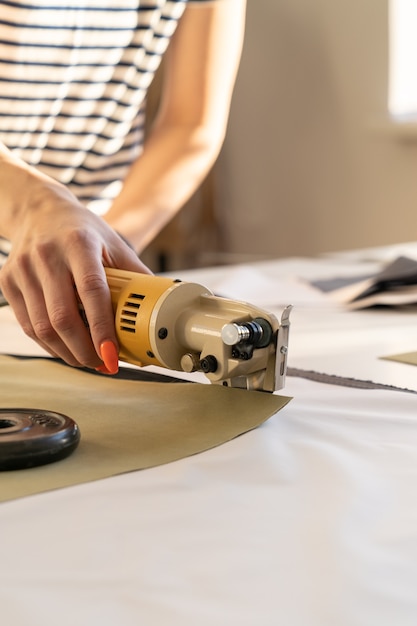In this professional, slightly out-of-focus image, a woman is seen working at a table covered with fabric. She holds a motorized fabric-cutting device with a yellow handle and a tan metal piece protruding from the top. The focus is directed towards her hand and the device, emphasizing its usage in cutting precise shapes from the fabric. A pattern, possibly a piece of paper, is pinned to the fabric with a small iron-like weight similar to those used in barbells, ensuring it stays in place during cutting. The background shows additional pieces of patterns and fabric, suggesting a setting geared towards sewing or tailoring work. The overall impression is of a meticulous and organized workflow centered on cutting fabric with a specialized tool.